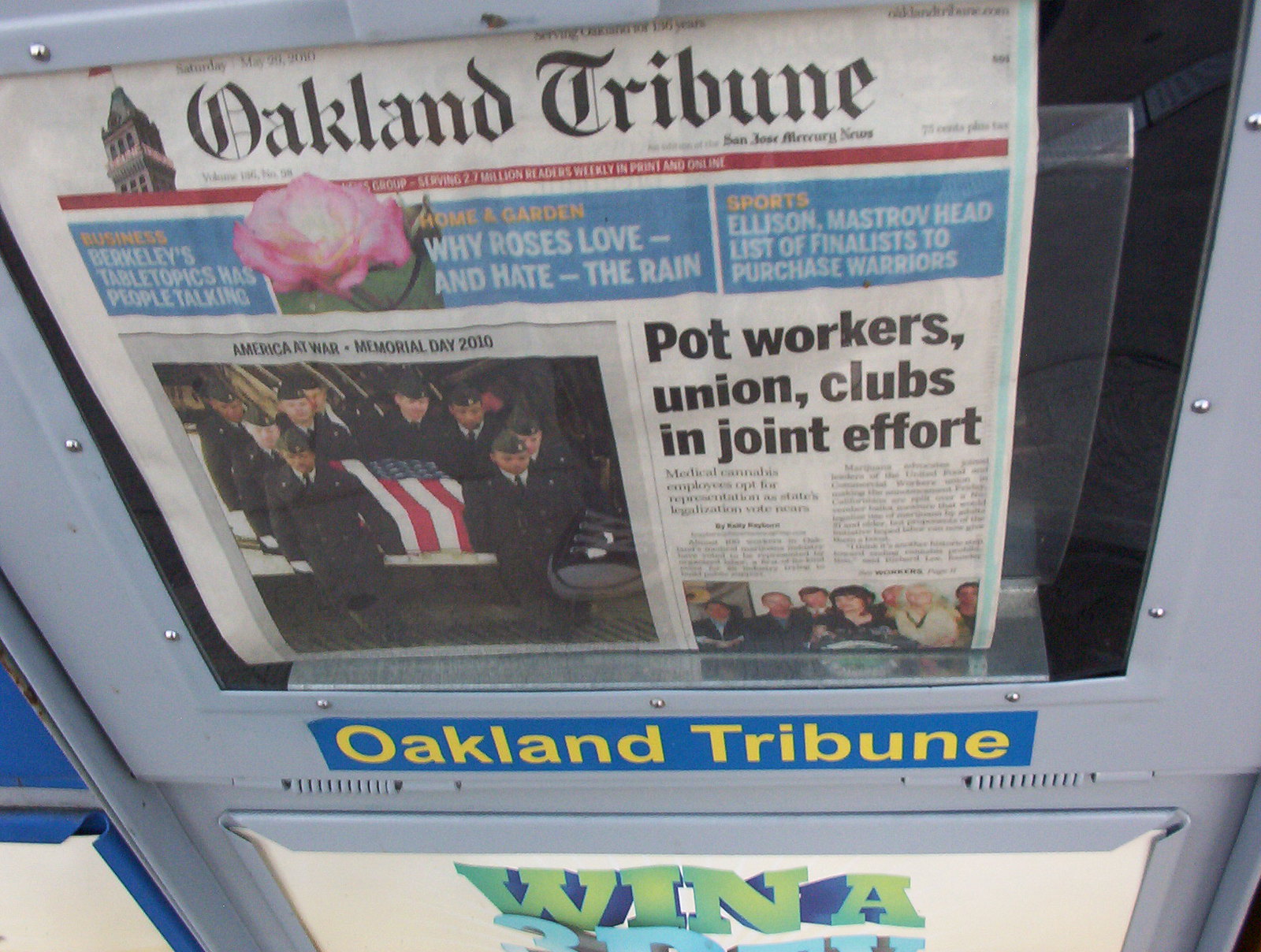This is an image of a gray newspaper box featuring the front page of the "Oakland Tribune." The newspaper box displays the words "Oakland Tribune" in yellow text against a blue background. Prominently visible on the newspaper front page is the headline "Pot Workers Union Clubs in Joint Effort." On the left side of the page, there's a poignant photograph of American soldiers carrying a flag-draped coffin, captioned "America at War Memorial Day 2010." Adjacent to the "Oakland Tribune" title on the actual paper, a clock tower is visible. Below the "Oakland Tribune" section on the box, the word "WINA" is written in a 3D-looking green font.